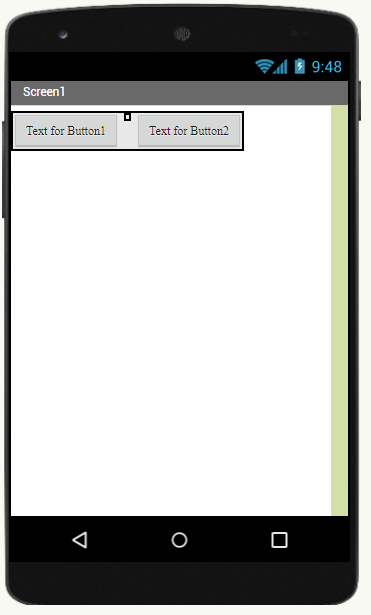This image depicts an older model mobile phone with a distinct, wider and shorter aspect ratio compared to contemporary devices. The phone features prominently large bezels, a characteristic thick chin, and forehead. At the top, the slightly curved and black bezel houses a centrally placed camera and another sensor slightly to the left. 

The bottom bezel contains three physical navigation buttons: a white back button on the left, a round central home button, and a square button on the right. The display shows various elements: 

- **Top-right corner**: Blue icons representing Wi-Fi, cellular signal strength, and battery life, with the time displayed as 9:48.
- **Top-left corner**: A grey bar containing white text "Screen 1."
- **Below the grey bar**: A white area with a green vertical bar on the far right edge.

In the center of the screen is a black-edged rectangle containing two smaller grey-edged rectangles with grey backgrounds. These rectangles are labeled "text for button 1" and "text for button 2," suggesting editable options. Between these two elements, there is a connector symbol, indicating a functional link or interaction between the two buttons.

Additionally, there is a small slider button on the left edge of the phone, likely for menu navigation or volume control. The screen appears to be displaying a setup or configuration interface, though the exact purpose is unclear.